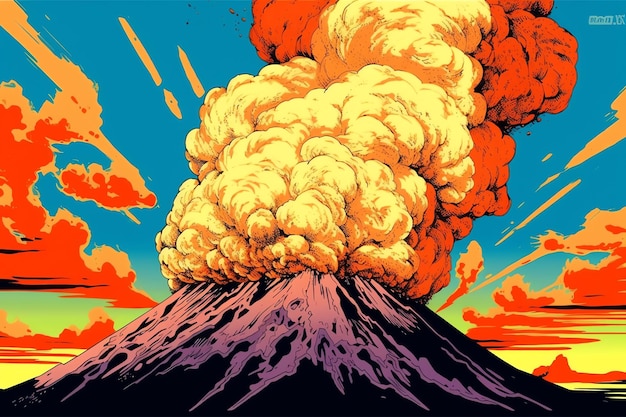This digital illustration, rendered in a comic book or cartoon style, vividly captures a volcano’s dramatic eruption. The volcano’s base is cloaked in black and muted lilac tones, giving it a dark, foreboding presence, while its apex spews forth an abundance of bright orange, red, and yellow smoke. This smoke has a uniquely puffy, cloud-like appearance, almost reminiscent of blossoming fungus, and billows upwards into a dynamically colored sky. The sky itself is a vibrant shade of blue, interspersed with striking orange and yellow clouds that seem to merge with the explosion, creating an almost surreal, flame-like effect. The overall scene is highly stylized, evoking the dramatic and abstract qualities typical of progressive rock album art. In the upper right corner, there is some unreadable text, adding to the illustration’s enigmatic allure.